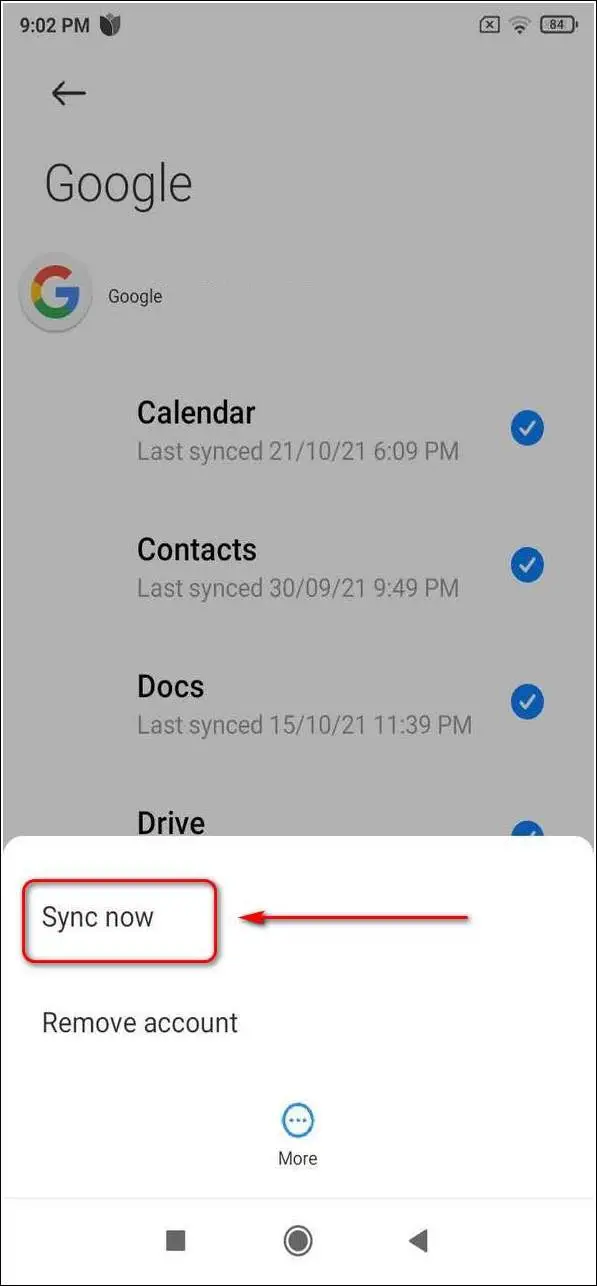This image is a smartphone screenshot of a Google synchronization settings page, captured at 9:02 PM. The status bar at the top of the screen shows a flower icon, a Wi-Fi symbol, and the battery level at 84%. There is a left-facing black arrow at the top left of the screenshot.

The page itself features a subtle gray overlay, with the word "Google" in black text, followed by the colorful Google "G" logo, and then the word "Google" again to the right. Below this header, various synchronization options are listed vertically:

1. **Calendar** - Last synced on October 21, 2021, at 6:09 PM, indicated by a white checkmark inside a blue circle.
2. **Contacts** - Last synced on September 30, 2021, at 9:49 PM, also denoted by a white checkmark in a blue circle.
3. **Docs** - Last synced on October 15, 2021, at 11:39 PM, marked by a white checkmark within a blue circle.

Beneath these entries is the **Drive** sync option, which also has a white checkmark in a blue circle. However, the text detailing its last synchronization time is obscured by a white pop-up box.

Within the white pop-up box, there is a red-outlined button labeled "Sync Now," with an arrow pointing to it from the right. Below this, there is black text stating "Remove Account." Additionally, at the bottom of the screen, there are buttons for "More," "Stop," "Home," and a left-facing arrow.